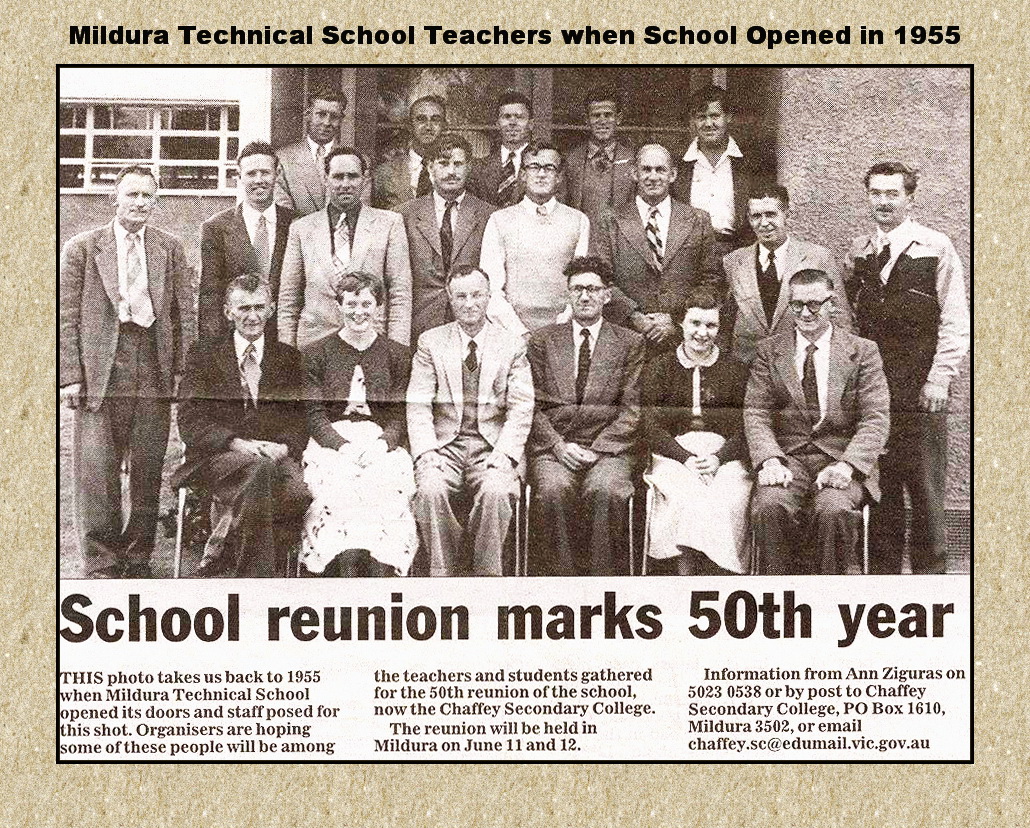The image is a vintage black and white photograph from a newspaper or publication, set against a beige background with visible fibers, resembling construction paper. The photograph, rectangular and in landscape orientation, shows staff members from Mildura Technical School when it opened in 1955, with a headline above stating "Mildura Technical School Teachers when school opened in 1955". The group consists of about 15 individuals arranged in three rows—a combination of men in suits and ties, and two women in skirts and cardigans seated in the front row on chairs. The men stand both in the middle and back rows. The accompanying text at the bottom mentions, "School reunion marks 50th year," providing details about a school reunion event for the now Chaffee Secondary College, set to take place in Mildura on June 11th and 12th, with contact information for Anne Zaguras for more details.